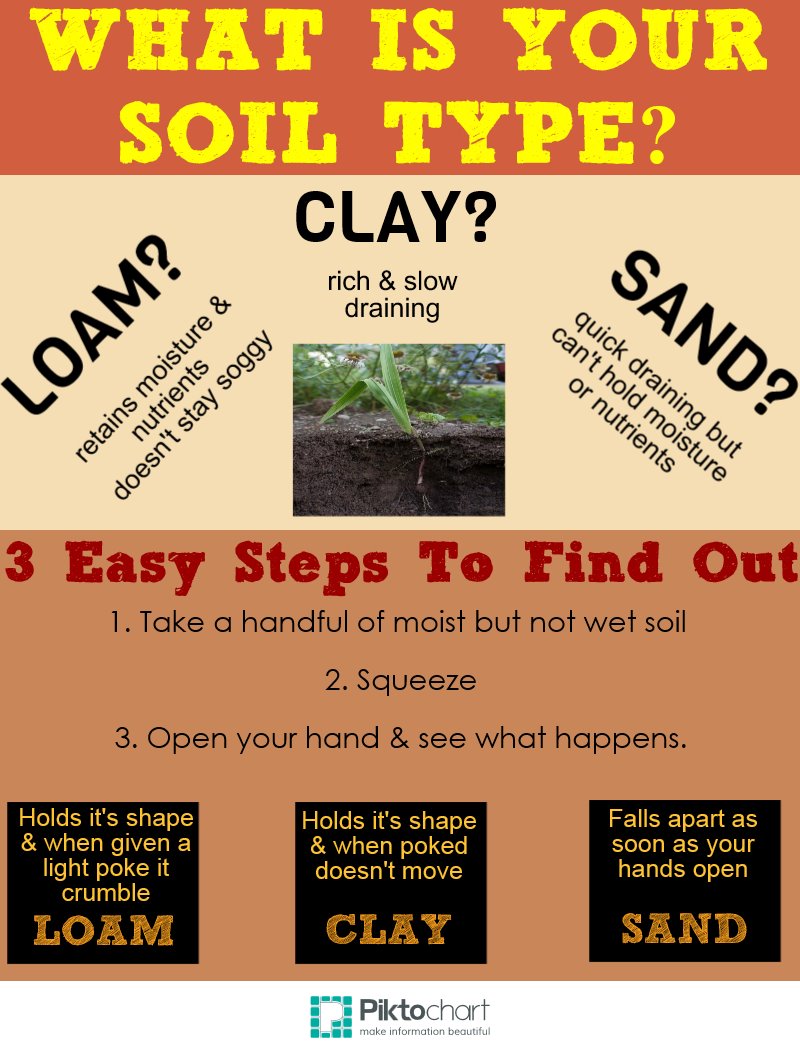The image features a detailed vertical chart with a tan and orange background, accentuated by yellow letters at the top asking, "What is your soil type?" Below this, in black text, it lists the possible soil types: loam, clay, or sand. Central to the chart is a small illustration of soil with plants growing from it, visually highlighting the topic.

At the bottom, in red text, the chart promises "Three Easy Steps to Find Out." In black text, these steps are laid out as follows:
1. Take a handful of moist but not wet soil.
2. Squeeze.
3. Open your hand and observe the results.

The chart also provides information on interpreting these results:
- **Loam**: Retains moisture and nutrients, doesn’t stay soggy. If the soil holds its shape when lightly poked and then crumbles, it's loam.
- **Clay**: Rich in nutrients but slow-draining. If the soil holds its shape when poked and doesn't crumble, it's clay.
- **Sand**: Quick-draining but poor at holding moisture and nutrients. If the soil falls apart as soon as you open your hand, it's sand.

In the footer, the chart announces, "Make information beautiful" and offers brief explanations of the three soil types, reaffirming the earlier descriptions.